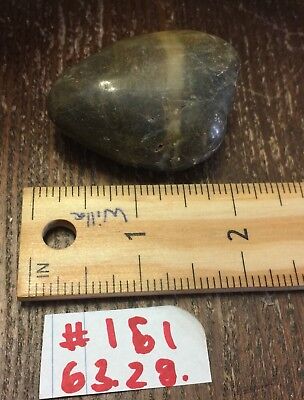The photograph captures a section of an old, dark wooden desk surface, characterized by visible grain and lighter tan scratches indicative of age and use. Centrally positioned in the image is the end of an unusual wooden school ruler, showing only the first two and a half inches. This ruler features its numbers aligned down the middle rather than along the edge, and has "Willa" or "Willie" written on it, possibly in pencil. Below the ruler, there is a piece of lined notebook paper, seemingly torn from a college-ruled notebook, with the handwritten inscription "#16163.28" in red marker, resembling the handwriting of a child. Above the ruler lies a polished gray pebble, approximately two inches long, with a distinctive lighter gray stripe encircling it, possibly a mineral specimen or a precious stone.